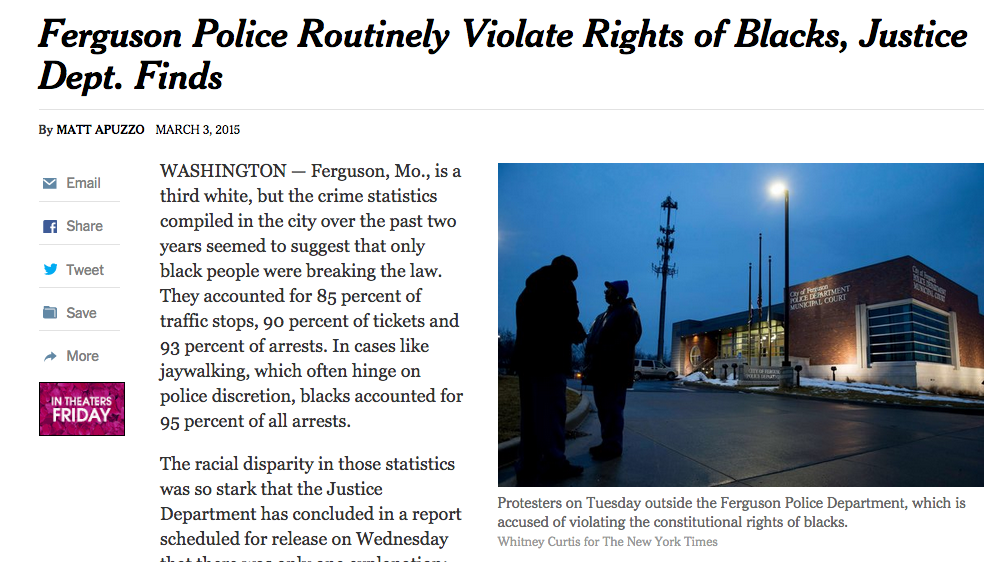The image is a color, landscape-format screenshot from an online news article. The headline reads "Ferguson Police Routinely Violate Rights of Blacks, Justice Department Finds," authored by Matt Apuzzo and dated March 3rd, 2015. The article opens with the location Washington and reports on findings from Ferguson, Missouri. It describes how, although Ferguson is one-third white, crime statistics from the past two years suggest disproportionate law enforcement against black individuals. Specifically, black individuals accounted for 85% of traffic stops, 90% of tickets, and 93% of arrests. In discretionary cases like jaywalking, blacks made up 95% of all arrests. The data's stark racial disparity led the Justice Department to conclude in a report set to be released on Wednesday, although the text below this point is illegible due to the image cut-off.

To the right of these paragraphs, there is a photograph of two protesters outside the Ferguson Police Department, which has been accused of violating the constitutional rights of black residents. These individuals are engaged in conversation in the parking lot. The caption beneath this image identifies them as protesters from Tuesday.